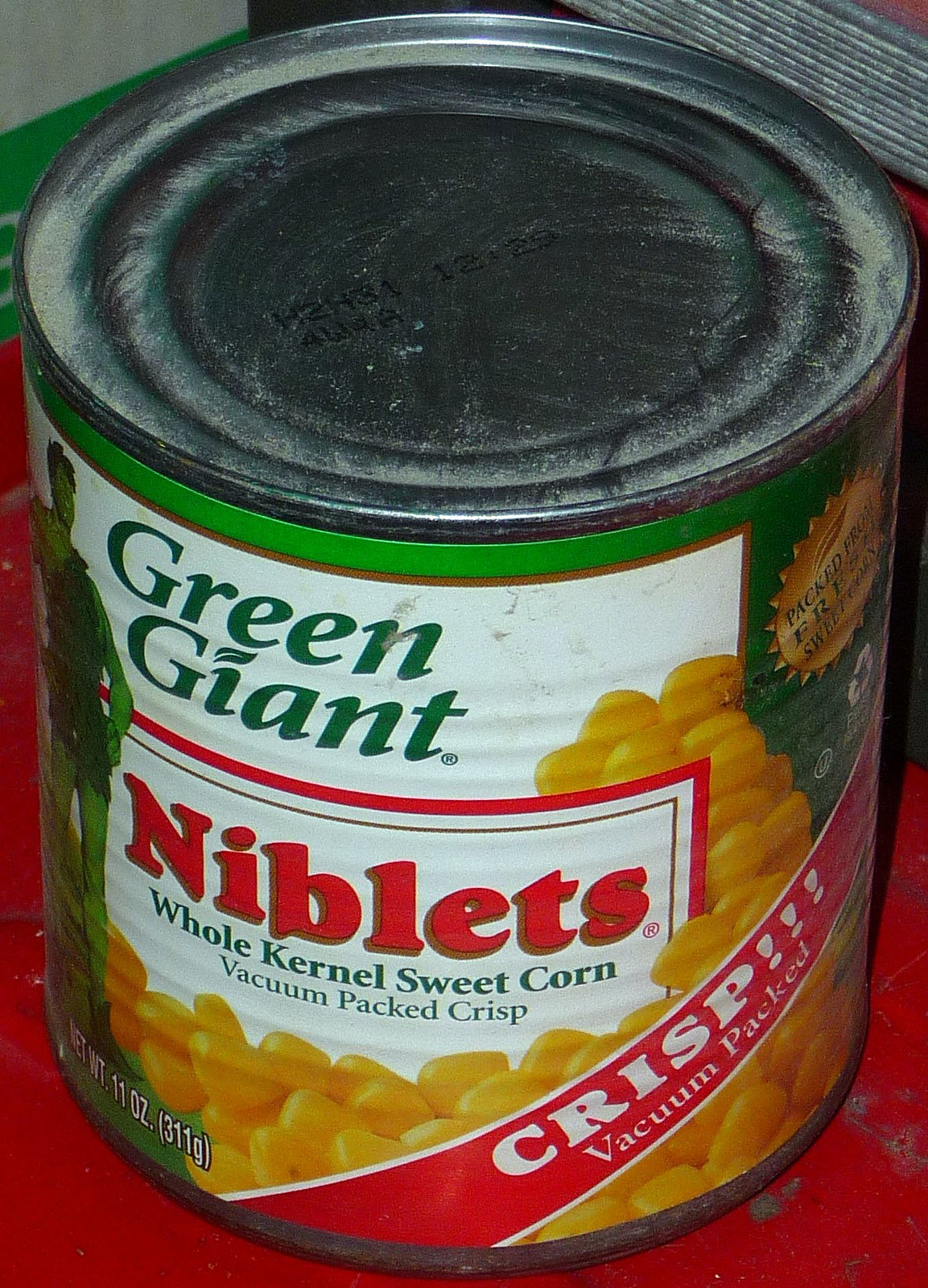The image showcases a can of Green Giant Niblets Whole Kernel Sweet Corn resting on a weathered red table. The can, displayed at an angle from above, reveals both the top and a portion of the front, giving it a tilted appearance towards the viewer. The iconic Green Giant character and logo are prominently visible, along with the product name "Niblets" in bright red lettering. The label features an appetizing picture of yellow corn and specifies that the can contains 11 ounces (311 grams) of corn. Additionally, a diagonal banner across the can reads "Crisp, Vacuum Packed."

The red table underneath the can is visibly marked, with chipped paint and indications of dirt, adding a rustic feel to the scene. Behind the can, a vertical wall showcases an alternating pattern of pale green and dark green bands, with a white section above. This backdrop also displays signs of wear, with chipped and marked paint. At the level of the can's top, a metal band with horizontal detailing is visible. The top of the can itself appears dusty, dirty, and exhibits some scratches. The lighting in the image is concentrated on the area that highlights the word "Niblets."